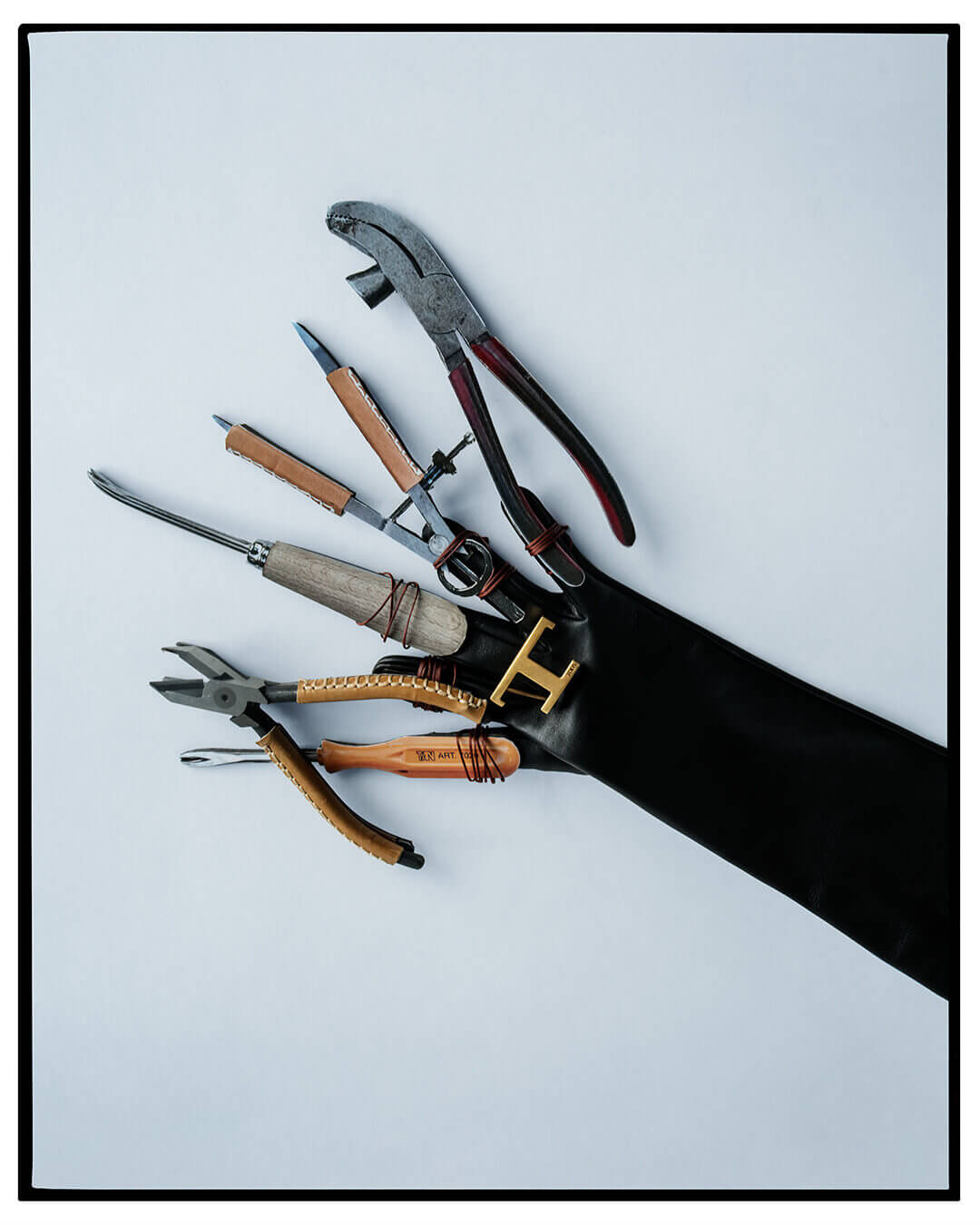The image is an artistic rendition of a black glove designed to look like a human hand, extending all the way up the arm. The glove separates into five distinct fingers, each uniquely equipped with a different tool, intricately attached to each finger. The thumb features a screwdriver, while the index finger has a pair of clippers or tweezers. The middle finger is affixed with a small handheld pick or ice pick. The ring finger has a compass, attached with a red rope or wire, adding a touch of color to the monochromatic glove. Finally, the pinky finger supports a pair of pliers. The black rubber of the glove contrasts sharply with the metallic and functional appearance of the tools, creating a striking visual blend of utility and artistry.